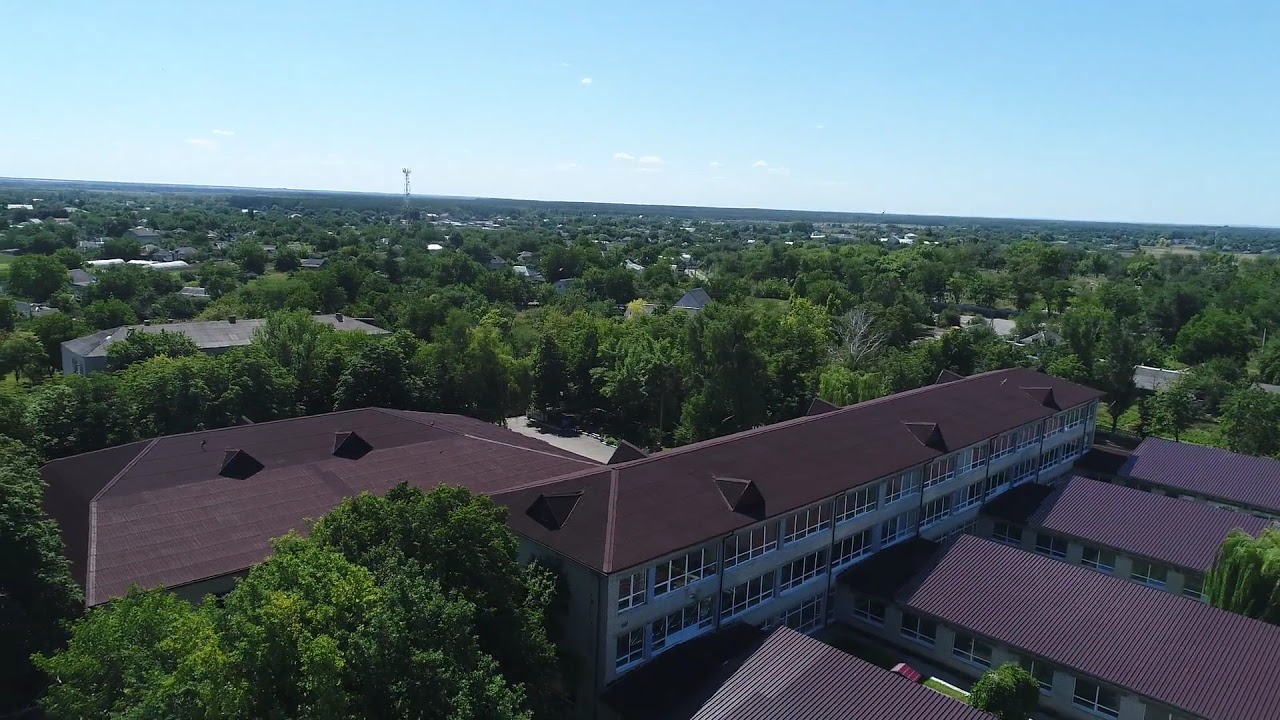This aerial photograph captures a scenic view from approximately 100 feet above the ground on a bright, sunny day with few clouds. The central focus is a cluster of large buildings tightly surrounded by tall, green trees, giving the impression that this area is nestled in a forested environment. The most prominent building is a narrow, long structure with a sloped, dark brown roof, stretching six times longer than it is wide, and featuring 20 to 30 windows along its length. Perpendicular to this, there is a slightly taller building with a similar slanted roof and rows of windows, distinguished by small out-peaks on its roof. Nearby, another building shares the same roofing style but is wider and shorter. Behind these central structures, additional rooftops emerge from the treetops, hinting at further development. In the distance, more buildings and trees can be seen, along with a radio or cell phone tower standing out near the center of the image. The sky above is a bright blue with minimal white glare from the sun, adding to the overall tranquil and picturesque atmosphere of the scene.